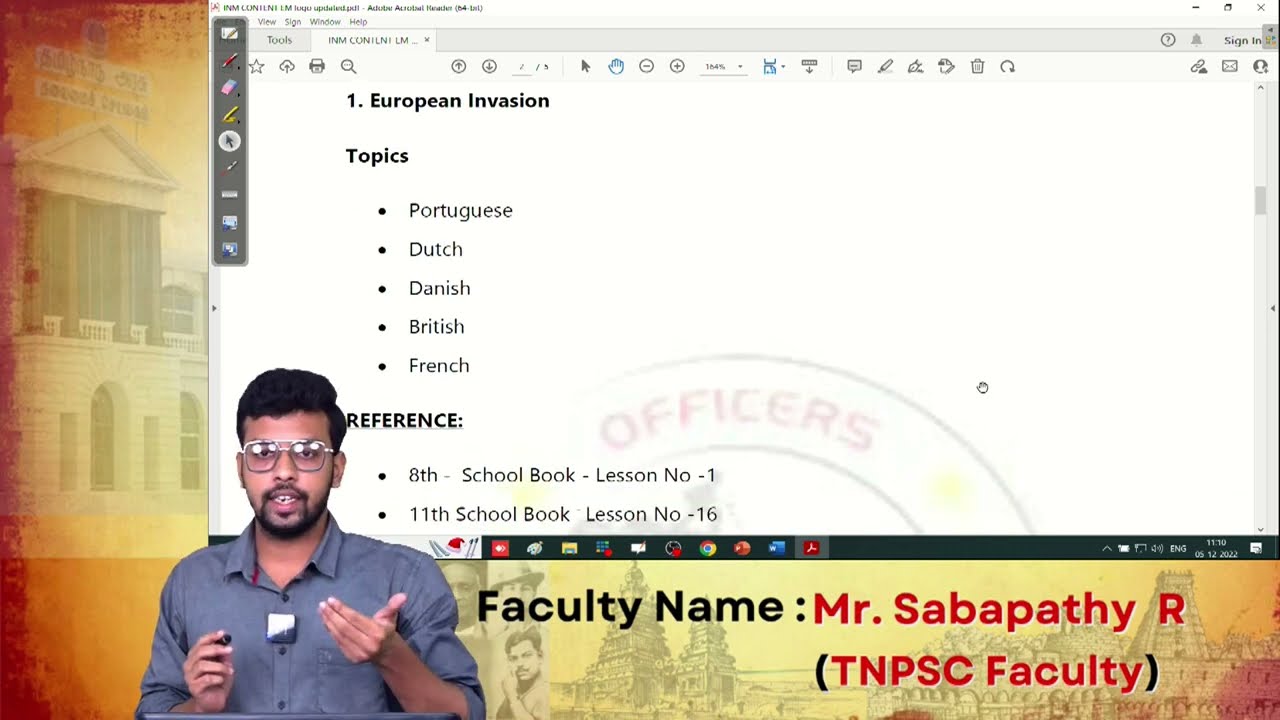The image showcases an Indian professor named Mr. Sabapathy, who appears to be giving a presentation. He has a neatly trimmed black beard, poofy black hair, and is wearing glasses along with a blue button-down shirt with the sleeves rolled up. He is gesturing with his hands, suggesting an active explanation. 

In the background, there's a slide projected on what looks like a Windows screen. The slide is written in a plain font and includes the following topics: European invasion, with specific focus on Portuguese, Dutch, Danish, British, and French. Below these topics, there are references to "8th school book, lesson no. 1" and "11th school book, lesson no. 16". Additionally, it lists "Faculty name: Mr. Sabapathy, R." with "TNPSC faculty" in red text and the rest in black. 

The setting behind the screen shows buildings that resemble memorial or government structures, adding an academic or formal atmosphere to the scene. The intricate details of his appearance and the text on the screen imply a thorough and structured teaching session, possibly an overview of a syllabus related to European invasions.